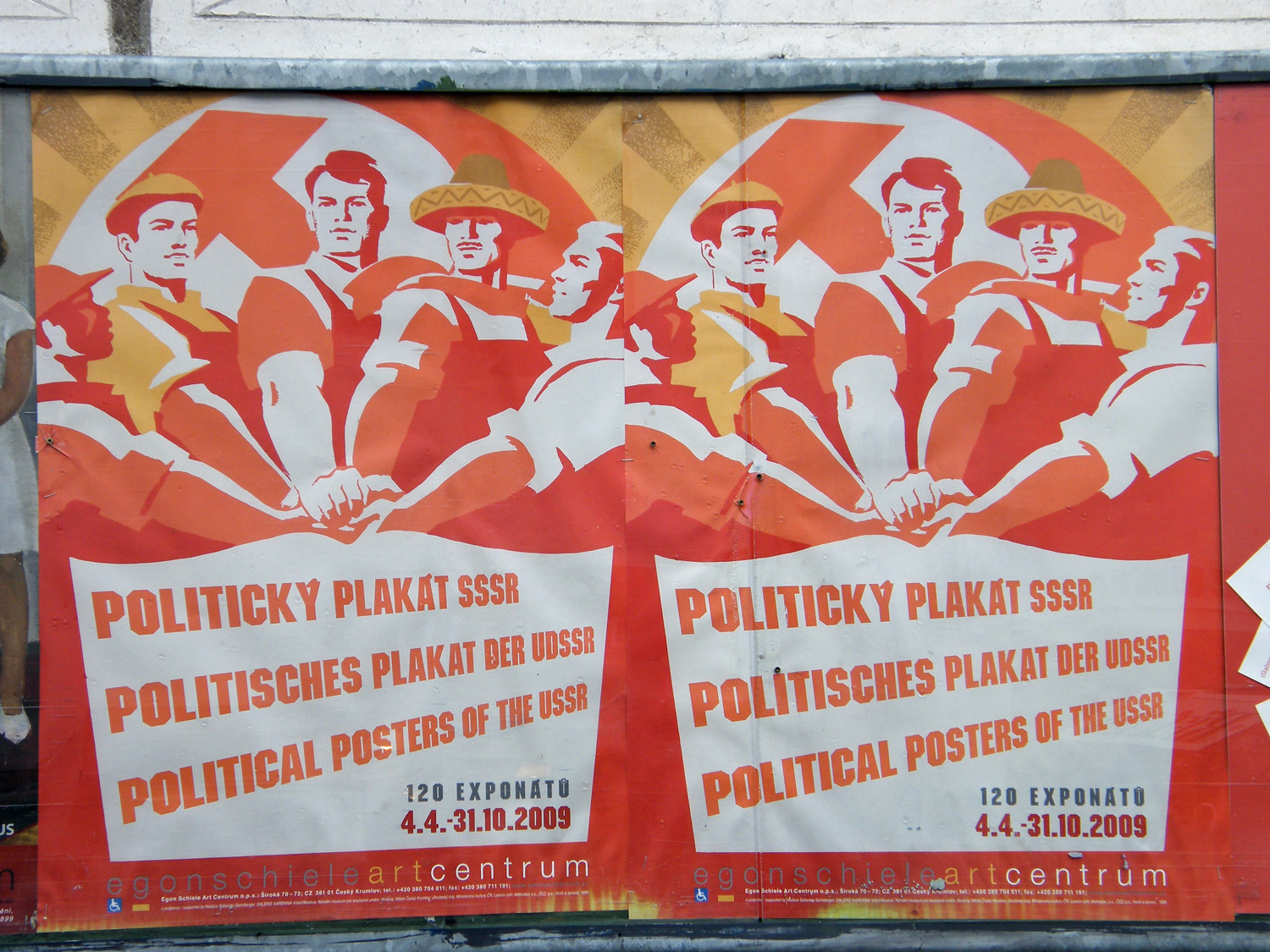The image depicts two identical posters side by side, primarily in vibrant hues of red, orange, and yellow. Each poster features five laborers, likely blue-collar or farming-types, standing in a circle with their hands joined in the center, reminiscent of a post-huddle gesture. The background prominently displays the Soviet emblem, the hammer and sickle. The main text on the poster, translated into multiple languages including German, Czech, and English, reads "Political Posters of the USSR." Additional text in the bottom right corner states "120 Exponatu, 4.4 - 31.10.2009," suggesting it is an art exhibit organized by the Egon Schiele Artszentrum. The posters evoke a sense of solidarity among workers, potentially alluding to the slogan, "Workers of the World, Unite."